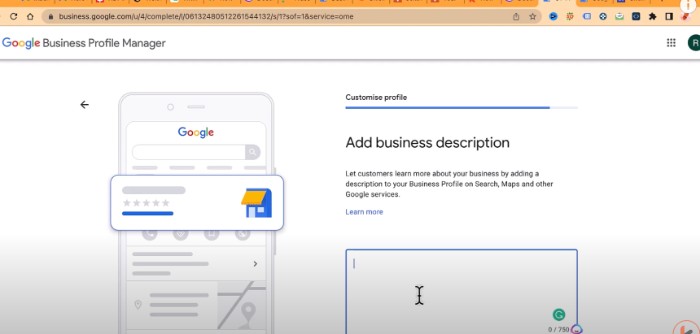Displayed on a computer screen is a webpage titled "Business Profile Manager," observable at the URL business.google.com, entered into the browser's search bar. Dominating the page is the familiar "Google" logo in its bright, multicolored design. Below the logo, there is a large pop-up featuring a graphic that appears to be either a mailbox with something emerging from it, or a building adorned with an awning. This illustration is accompanied by a series of hollow, gray stars, likely intended as a rating system, and a similarly gray, unused search bar. A solid blue progress bar is situated beneath these stars, indicating some level of completion.

Adjacent to this graphic, in bold black text, is the option "Customize Profile," with an accompanying progress bar that's approximately 7/8ths filled, signifying near-completion. Below this, users are prompted to "Add a Business Description," emphasized by a clickable "Learn More" link in blue font.

Further down the page, there is a white rectangle bordered in blue. Within this, a pair of black brackets is displayed, connected to a green circle emblazoned with a "G," likely representative of a Google-related feature or tool. This detailed layout indicates a comprehensive and interactive platform for managing a business profile on Google.